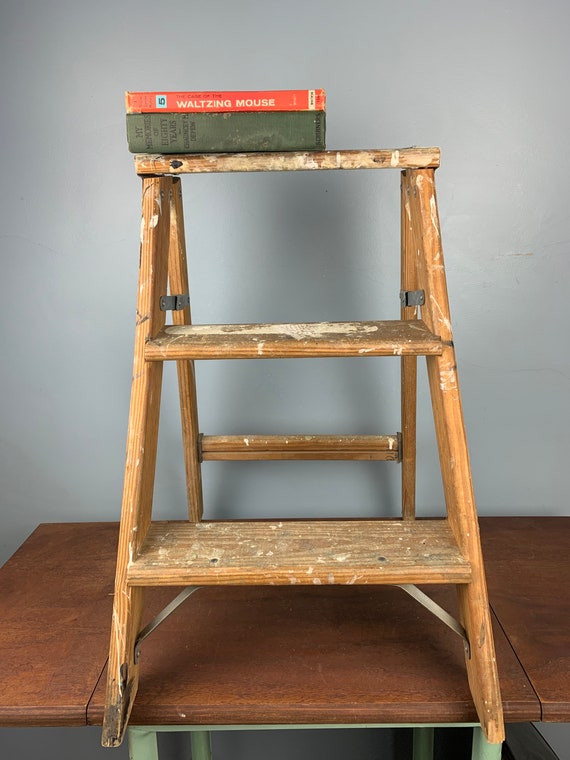In the color photograph, framed in portrait orientation, the primary focus is a well-worn, mid-brown wooden step ladder with two steps leading to a small platform at the top. This ladder is heavily splattered with creams and whites, likely paint and plaster, indicating extensive use. Facing the ladder head-on, you can observe black metal clasps riveted at the top to open the ladder, and additional similar-colored straps with light silver elements at the bottom.

The ladder stands on a dark oak table that runs horizontally across the image. The table, with three-leaf divisions extending from front to back, features green-framed legs that just peek into view where the image cuts off. On the left side of the top platform of the ladder rest two books. The upper book is red with the white text "Waltzing Maus" on the spine, while the one beneath it is darker, an indistinct gray-green, with barely visible horizontal text.

In the background, a light gray wall with some plaster imperfections on the right side adds character to the setting, making it less than perfect but more authentic. The ladder, table, and wall together create an organized yet artistic composition, possibly staged for a painting or photograph.